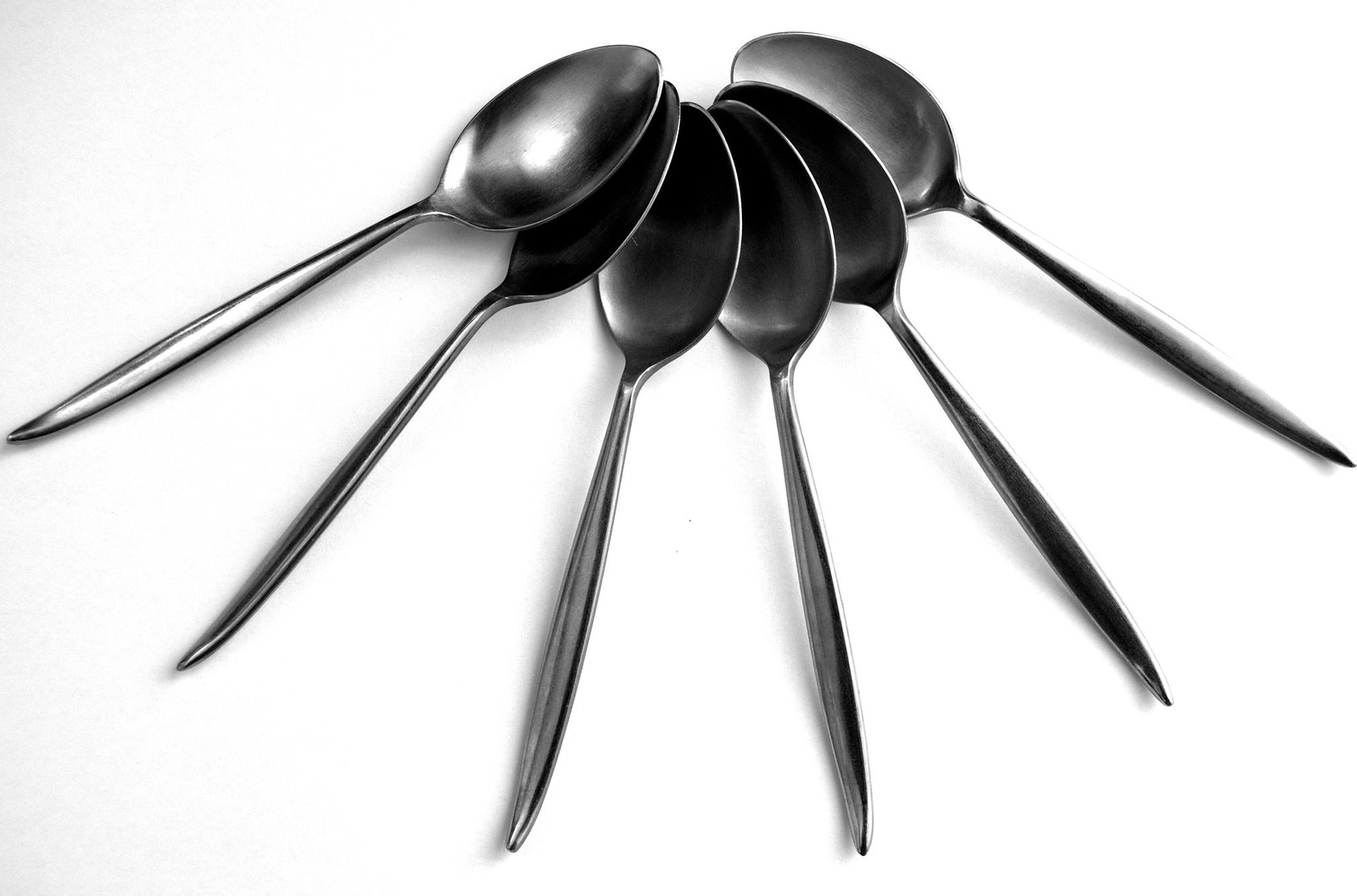This photograph showcases a meticulously arranged set of six soup spoons, each in a simple and elegant design. The silver spoons, with their brushed yet slightly polished finish, are stacked and overlapping in a semi-circle, creating a striking, spoke-like pattern with the handles radiating outward. Set against a gradient background that transitions from gray to white, the reflective quality of the spoons captures and plays with the light, particularly highlighting the spoon on the left. This setup emphasizes the clean lines and reflective surfaces of the spoons, which stand out against the solid, minimalistic backdrop. The scene is thoughtfully composed, with every handle extending uniformly, adding a sense of balance and symmetry to the overall arrangement.